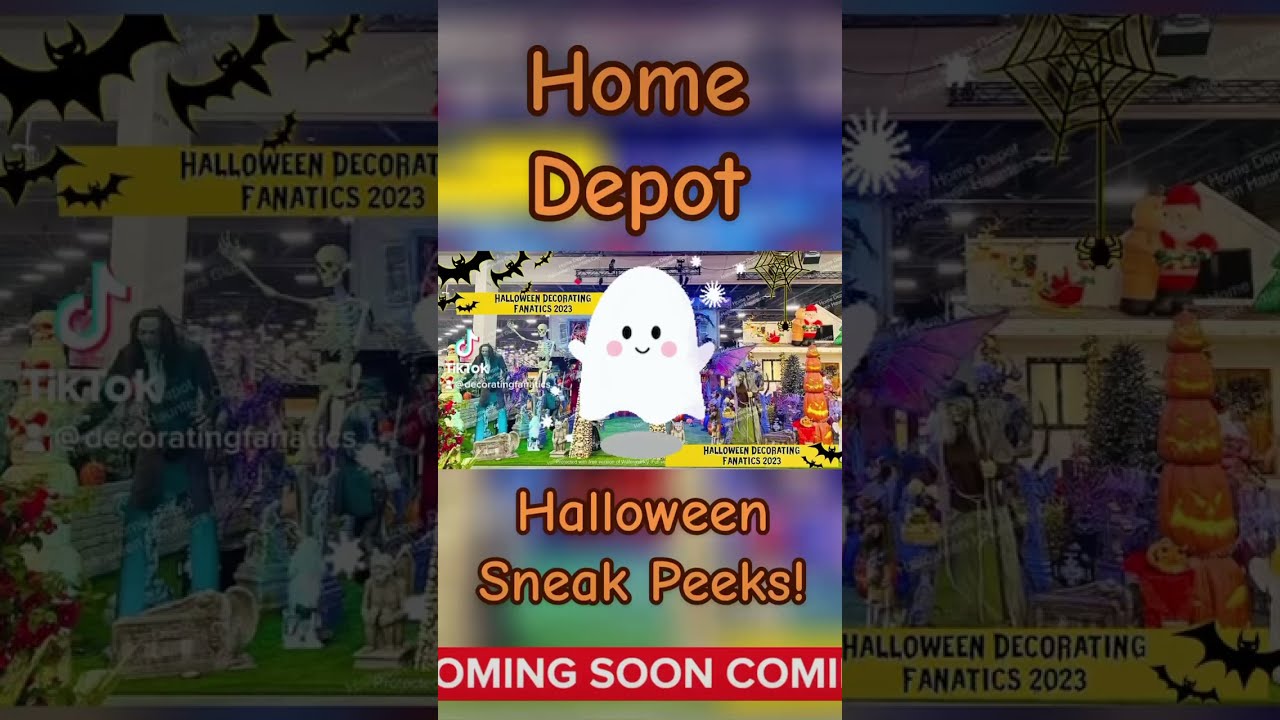The image is a screenshot of a TikTok advertisement promoting Home Depot's upcoming Halloween decorations for 2023. The main focus is a central, cell phone-style vertical video, flanked by blurred, zoomed-in extensions of the same image on either side. At the top of the screen, "Home Depot" is written in orange Comic Sans font with a red outline. Below this, the text "Halloween Sneak Peeks!" is displayed, with a red ticker tape at the very bottom reading "coming soon" in white letters. The central image shows a festive Halloween display with traditional characters such as a white ghost with pink cheeks and a smile, pumpkins stacked like a Christmas tree, skeletons, gravestones, gargoyles, cemetery figures, vampire bats, and spider webs. Interestingly, there's also a Santa Claus figure. Signs reading "Halloween Decorating Fanatics 2023" are visible in yellow with black font, located in the top left and bottom right corners of the Halloween display. The TikTok watermark is present, indicating the image is from the platform.